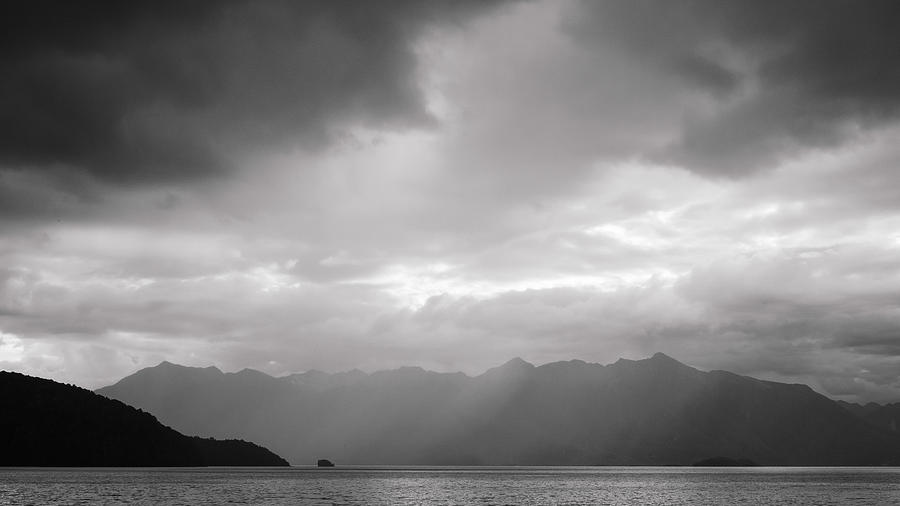This is a dramatic black-and-white photograph capturing a coastal landscape with a stormy ambiance. In the foreground extends a body of water, with delicate ripples touching the shoreline on the bottom left corner. Here, a dark, large hill with hints of vegetation slopes gently into the water, ending in a rock formation. The water stretches across the entire bottom of the image, from the left to the right.

Dominating the top two-thirds of the photograph is a heavily clouded sky, darkening ominously at the upper left and right corners. Despite the oppressive cloud cover, a sliver of light breaks through the center, casting rays and illuminating patches of the scene. This light reveals the rain falling softly over a distant, rugged mountain range, creating a misty atmosphere.

In the background, the rough silhouettes of mountains and hills appear in varying shades of gray and black, contributing to the monochromatic, moody tone of the photograph. The image captures a sense of serene yet powerful nature, with contrasts between light and dark, smooth water and jagged land providing depth and texture.